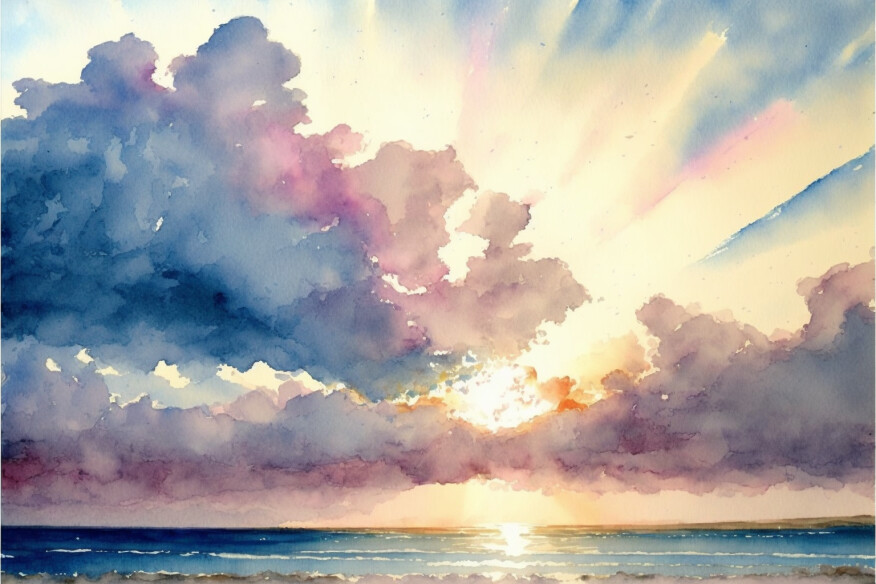This detailed hand-painted watercolor captures a serene sunset over the ocean. In the foreground, gentle waves ripple towards a faint shoreline at the bottom of the painting. Above, a glowing sun, partially obscured by long, branching clouds, casts a vibrant reflection on the water’s surface. The clouds, predominantly pink with hints of blue on the left, radiate outwards. The larger cloud in the bottom center extends to the left, leaving the right side of the sky mostly clear. The sky itself is a blend of pink, purple, gold, and yellow hues, with darker blues in the corners, especially the top right. The painting evokes a tranquil moment as sunrays softly illuminate the scene, highlighting the contrast between the warm, bright colors of the sunset and the darker tones of the clouds.